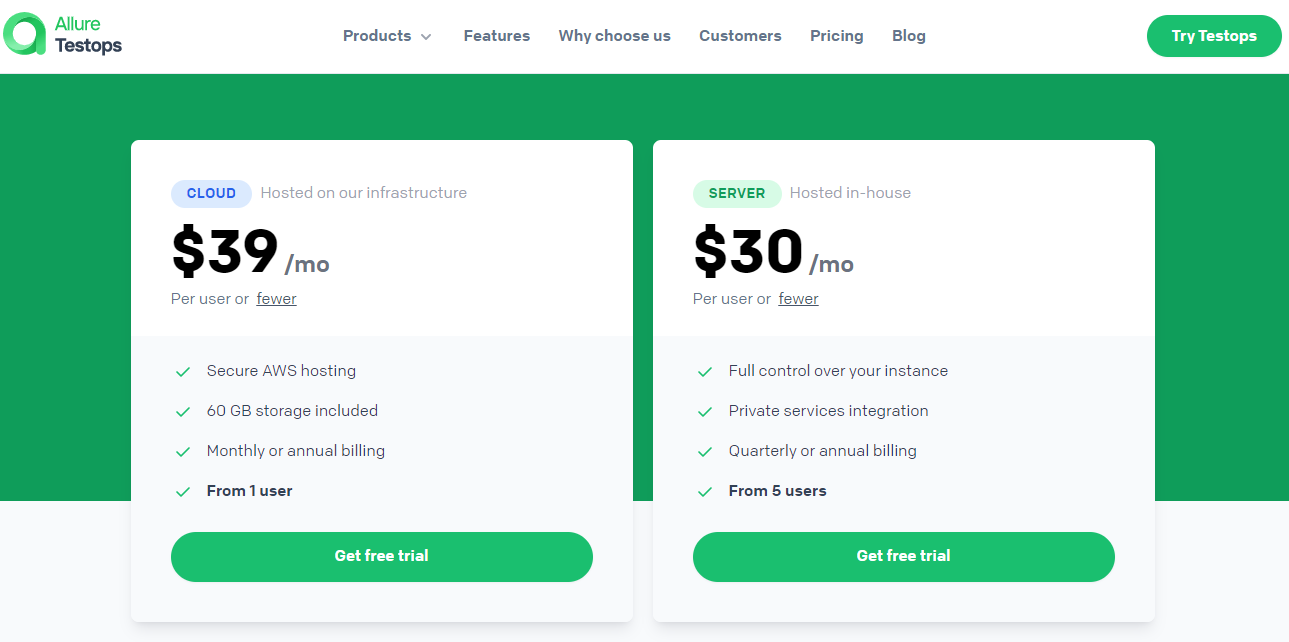Certainly! Here’s the cleaned-up and detailed caption:

---

The interface features a top-left icon, which is round and green, labeled “Allure Test Stops.” Centrally positioned at the top are several drop-down menus labeled: “Product,” “Features,” “Why Choose Us,” “Customers,” “Pricing,” and “Blog.” On the top-right, there's a prominent green button labeled “Try Test Stops.”

Below these elements, there's a horizontal green rectangular section with two white square panels. The left panel is light blue, titled “Cloud,” and includes the subtext: “Hosted on our infrastructure.” Beneath this, it states the pricing: “$39 a month per user or fewer.” Further down, there are four vertical checkmarks with corresponding descriptions: “Secure AWS Hosting,” “60 GB Storage Included,” “Monthly or Annual Billing,” and “Available from one user.” At the bottom of the panel, there's a green button labeled “Get Free Trial.”